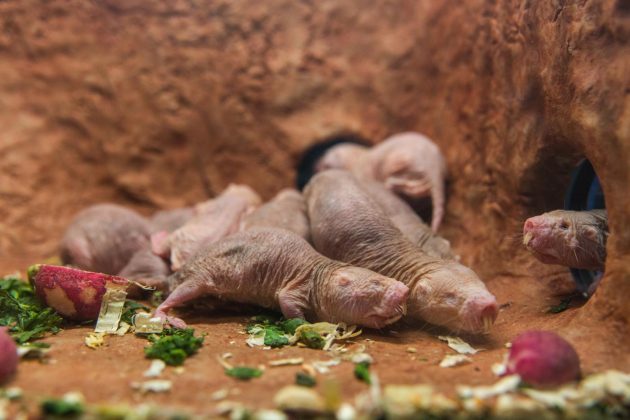In this detailed image, we're observing a den populated by several young, hairless creatures that appear to be either gophers or mole rats. They have distinctive features such as large front teeth and wrinkly, greyish skin that resembles leather. Most of these creatures seem to lack visible eyes, giving them a unique and somewhat eerie appearance. Their pinkish snouts and feet stand out against their otherwise grey bodies. The setting appears to be within a burrow, surrounded by reddish-brown sandy soil. Scattered around them are bits of vegetables with green leaves and dark red, possibly radishes or beets. In the foreground, two of these wrinkly creatures are in clear focus, while several more can be seen in the background and another pokes its head out from a tunnel on the right. Another tunnel in the back reveals yet another creature disappearing headfirst into it, adding to the sense of a busy, interconnected subterranean habitat. At the very bottom right of the frame, a small radish-like vegetable is also visible, emphasizing the presence of these food items within the scene.